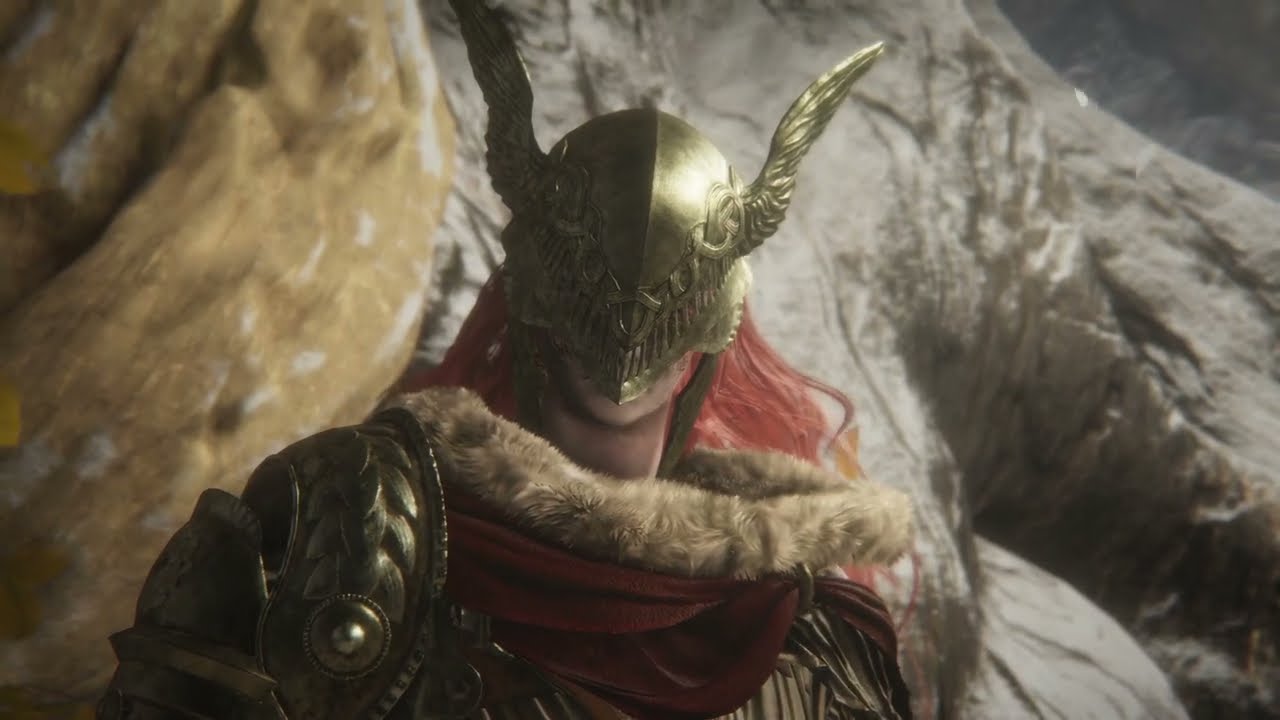This horizontal rectangular close-up image features a figure reminiscent of a Norse warrior or deity, possibly from a video game or movie. Central to the composition, the person has striking long red hair cascading around a full-face gold mask that comes to a V just above the chin, leaving only their neck and a portion of their chin visible. The mask, adorned with intricate slash marks over the eyes and nose area, extends into majestic gold wings at the sides, resembling eagle wings.

The figure's attire is richly detailed, with a light brown fur-lined cape snuggling around their neck. The fur is contrasted by a flowing red scarf beneath it, adding a vivid splash of color. Their armor includes a decorated dark gold or bronze guard on the right arm, while the left shoulder is protected by a robust, round, gold shield.

Set against a rugged backdrop of either tree trunks or rocky cliffs, the left side of the image features a brown hue, transitioning to a grayish tone on the right. This setting, void of greenery, enhances the raw, mythic atmosphere surrounding the warrior. The elaborate costume, with hints of medieval and Viking influences, combined with the natural, untamed background, paints a vivid scene of strength and ancient valor.